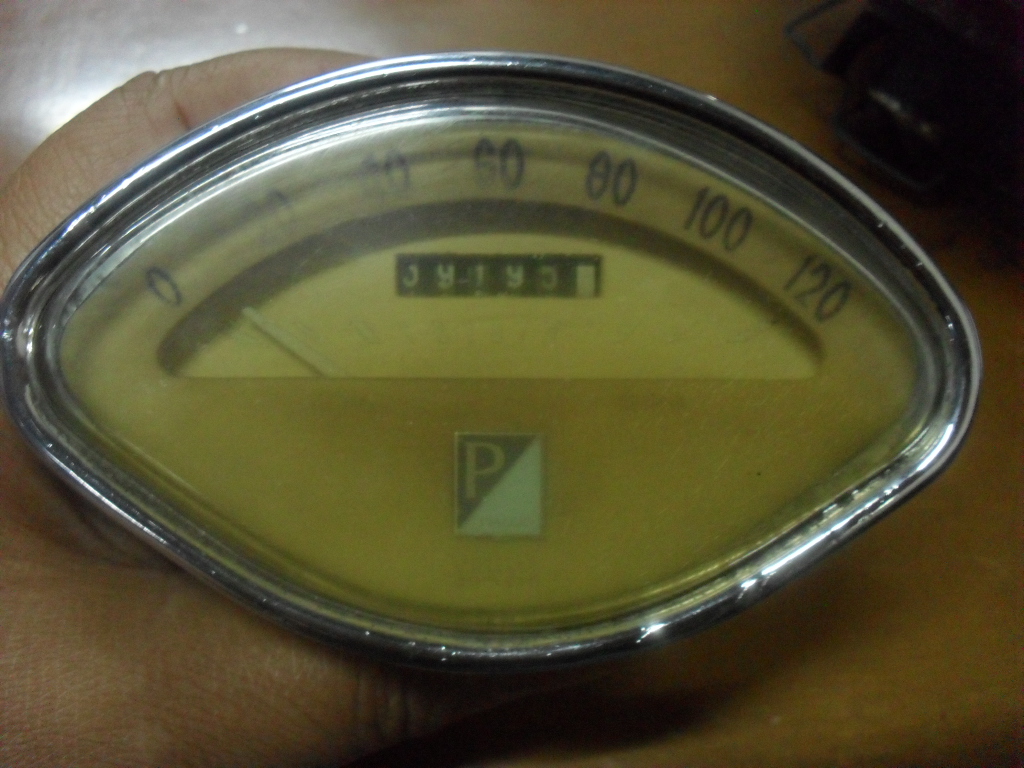The image depicts a close-up view of a hand, with visible fingers, holding a metallic speedometer. The speedometer features a black background with white numbers marking increments at 0, 20, 40, 60, 80, 100, and 120, indicating speed measurements. There is a white text, highlighted against the black background, though it appears to be upside down, making it difficult to discern its content. An arrow indicator on the speedometer points between 0 and 20, closer to the 0 mark.